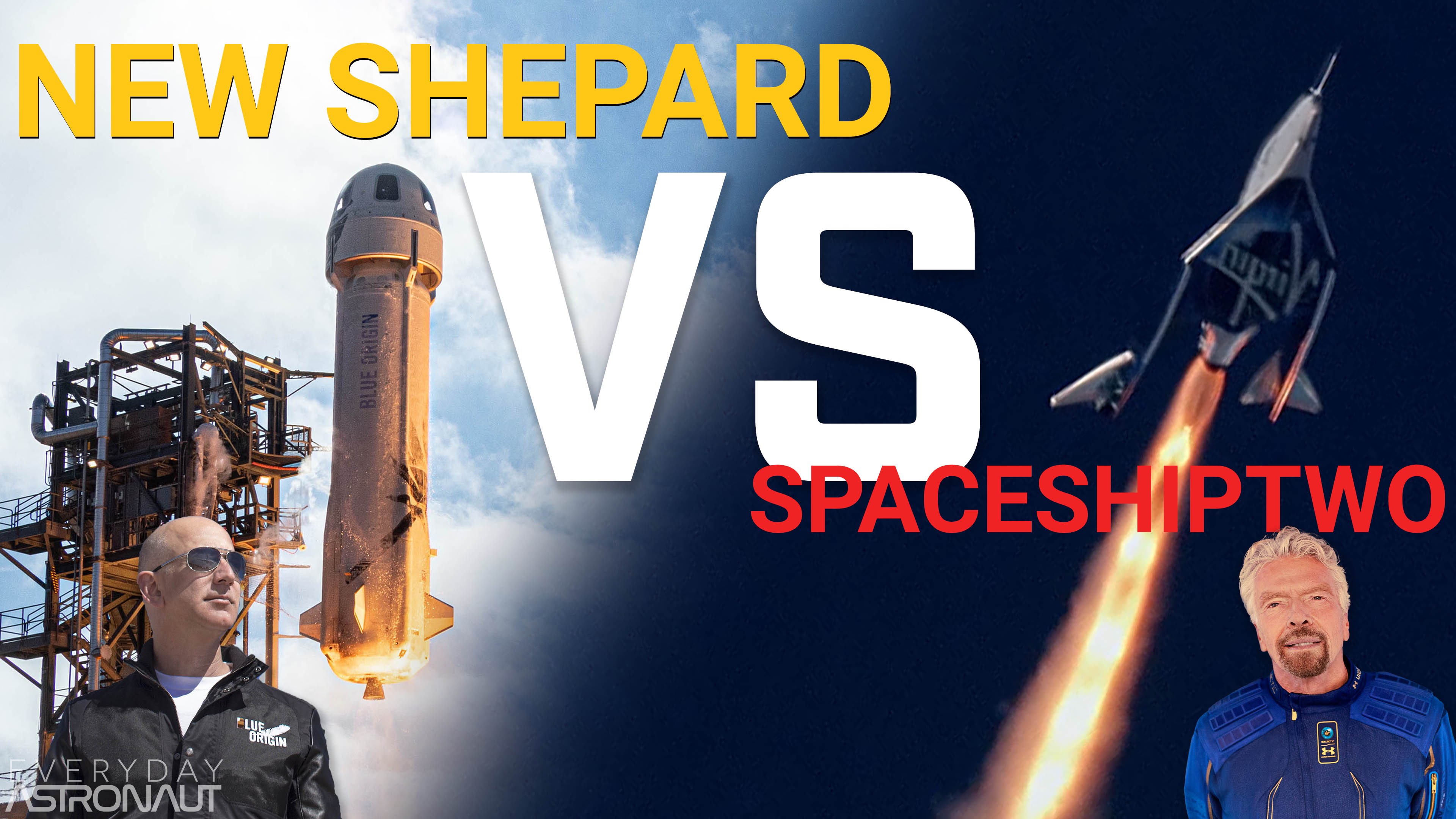This detailed image appears to be a video thumbnail depicting a comparison between two space missions. On the left side, the sky is blue with clouds, showcasing a rocket ship belonging to Jeff Bezos' "New Shepard," which is launching next to a tall structure. Jeff Bezos, identifiable by his bald head, aviator sunglasses, and black jacket, is standing beneath the rocket. To the left, at the top in large yellow text, it says "New Shepard."

In the center of the image, in bold, large white letters, the text "VS" stands prominently, dividing the two sides.

On the right side, the background shifts to a darker tone, with Richard Branson and his spacecraft. His rocket, bearing the Virgin logo, appears to be ascending into a darker sky, symbolizing space. Richard Branson is located in the bottom right corner, characterized by his white hair, goatee, and blue suit. Above him, in smaller red text, it states "Spaceship 2." The entire thumbnail effectively contrasts the two space endeavors with a feathered blend at the center, enhancing the visual distinction between the New Shepard and Spaceship 2 missions. The caption "Everyday Astronaut" appears prominently, connecting both sides of the graphic.